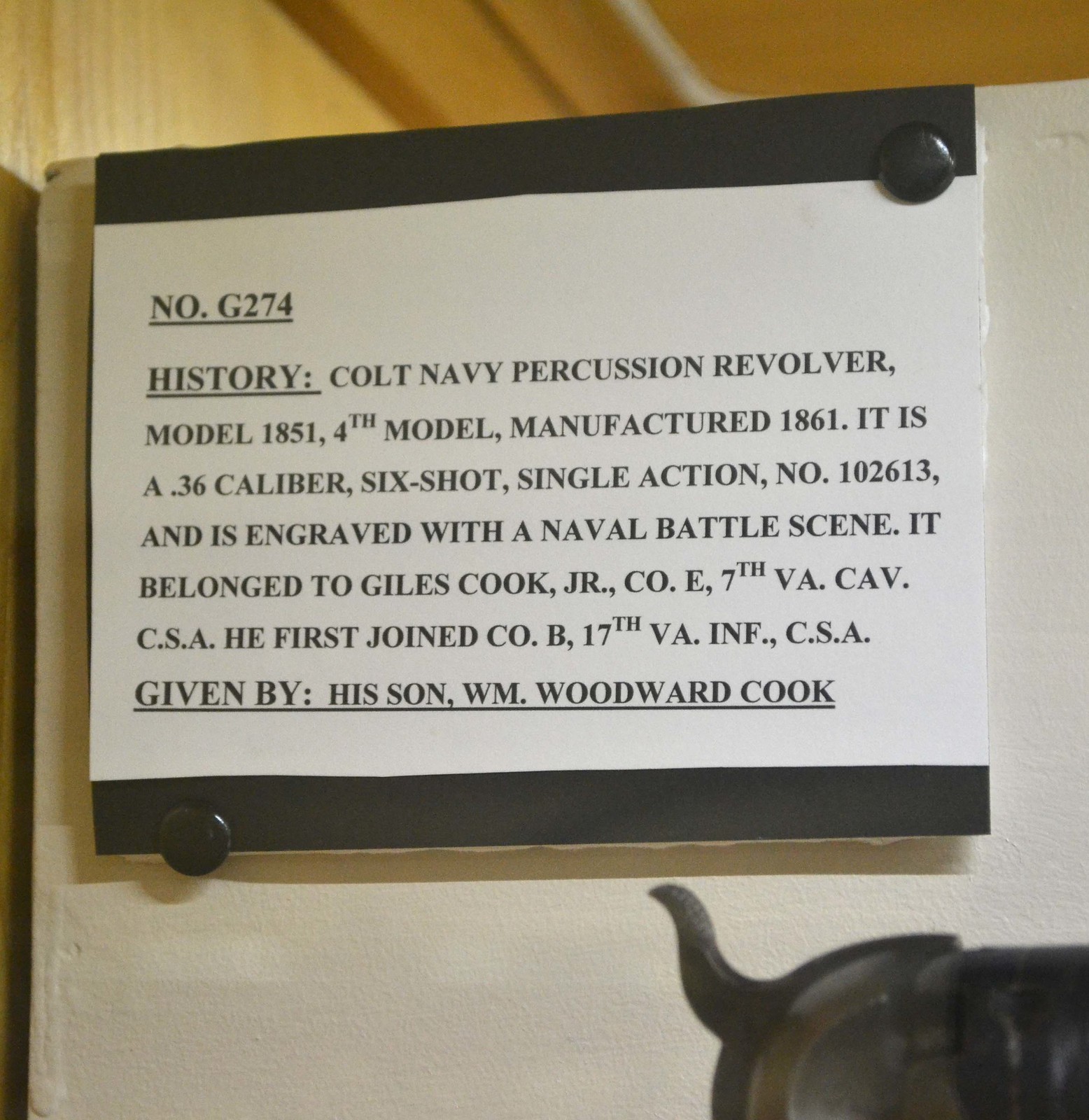This indoor photograph features a detailed sign mounted on a white board with black tacks, set against a backdrop of brown paneling. The top of the sign displays "G274" underlined, followed by "HISTORY" in capital letters, also underlined. The sign describes a Colt Navy Percussion Revolver, Model 1851, Fourth Model, manufactured in 1861. This .36 caliber, six-shot, single-action revolver, serial number 102613, is engraved with a naval battle scene. The revolver originally belonged to Giles Cook Jr., who served in Company E, 7th Virginia Cavalry, CSA, and initially joined Company B, 17th Virginia Infantry, CSA. The firearm was donated by his son, William Woodward Cook. In the bottom right corner of the image, part of the revolver itself is visible, showing the trigger and possibly a glimpse of the barrel.